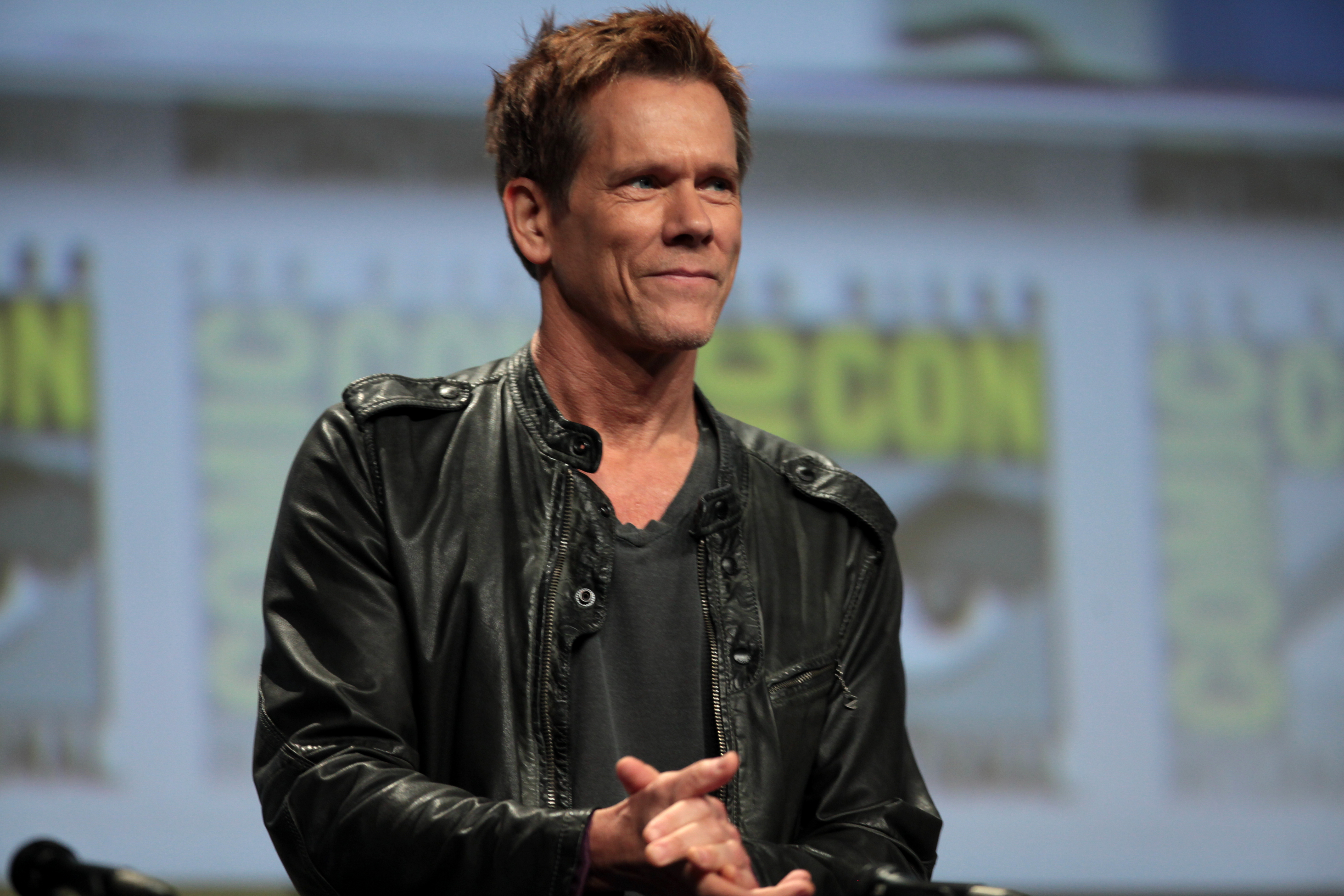In the image, Kevin Bacon stands at the center against a white backdrop featuring blurry text advertising Comic-Con in four different squares. Vertical and horizontal yellow lines mark the left and top edges of the background. Bacon is dressed in a black leather jacket with metal snaps at the top, worn over a well-used black t-shirt. His brown hair, uncombed and spiked in different places, contrasts with his very light eyebrows. He smiles softly, without showing his teeth, while looking forward and slightly to his left. His hands are clasped together in front of him, positioned below chest level. A microphone stands to his left, and subtle lines appear around his eyes, enhancing the depth of his smile. His eyes are blue, and his jacket appears slightly ruffled, adding to his casual yet charismatic presence.